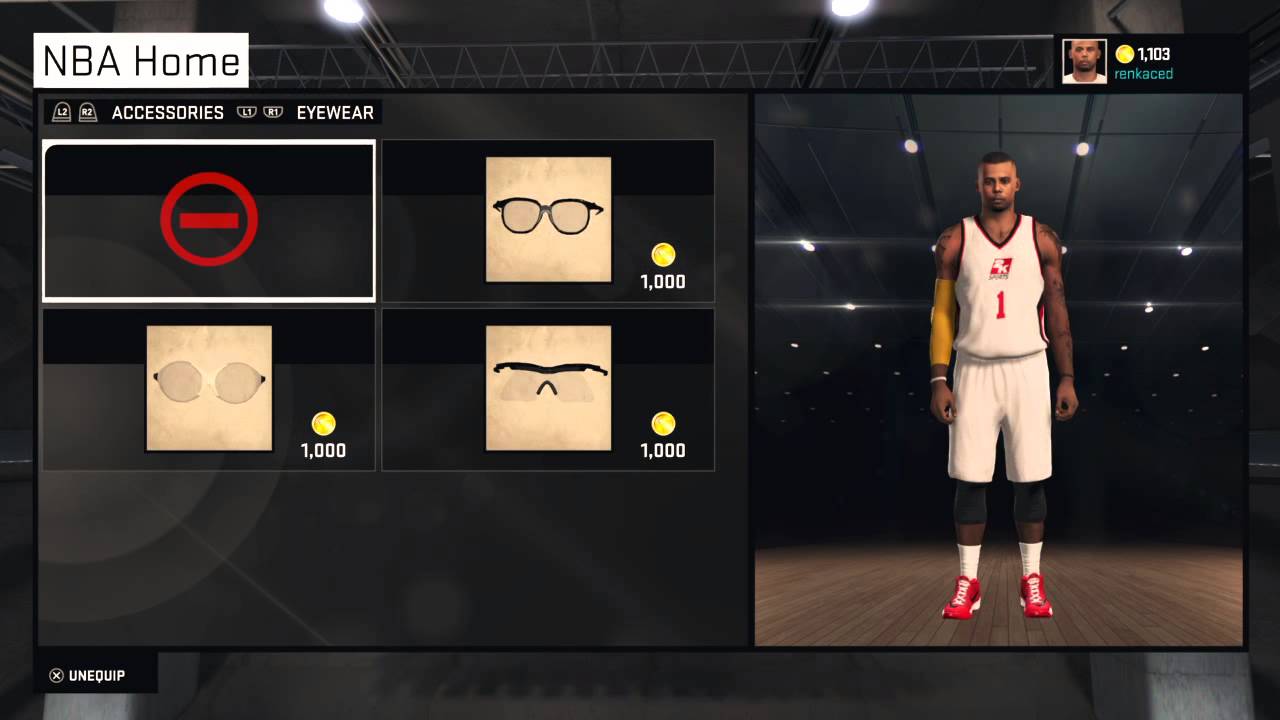In the image, a player is immersed in creating their character in the NBA 2K video game. The screen on the right showcases the character, a male with medium-dark skin tone and short hair, standing on a basketball court. He is dressed in a white jersey featuring the number "1" with "2K" inscribed above it, and accessorized with red sneakers, a compression sleeve on his right elbow, and multiple tattoos. Displayed at the top right is the gamer's tag, which appears to be "Ren Kaced," though it's slightly blurred and hard to discern. The player's in-game currency total is 1,103, visible next to the username. On the left side of the screen, there is a selection of accessories available for purchase, including glasses and goggles, each priced at 1,000 in-game currency. Among the options, some are standard eyewear, while others seem designed for sporting activities like biking.